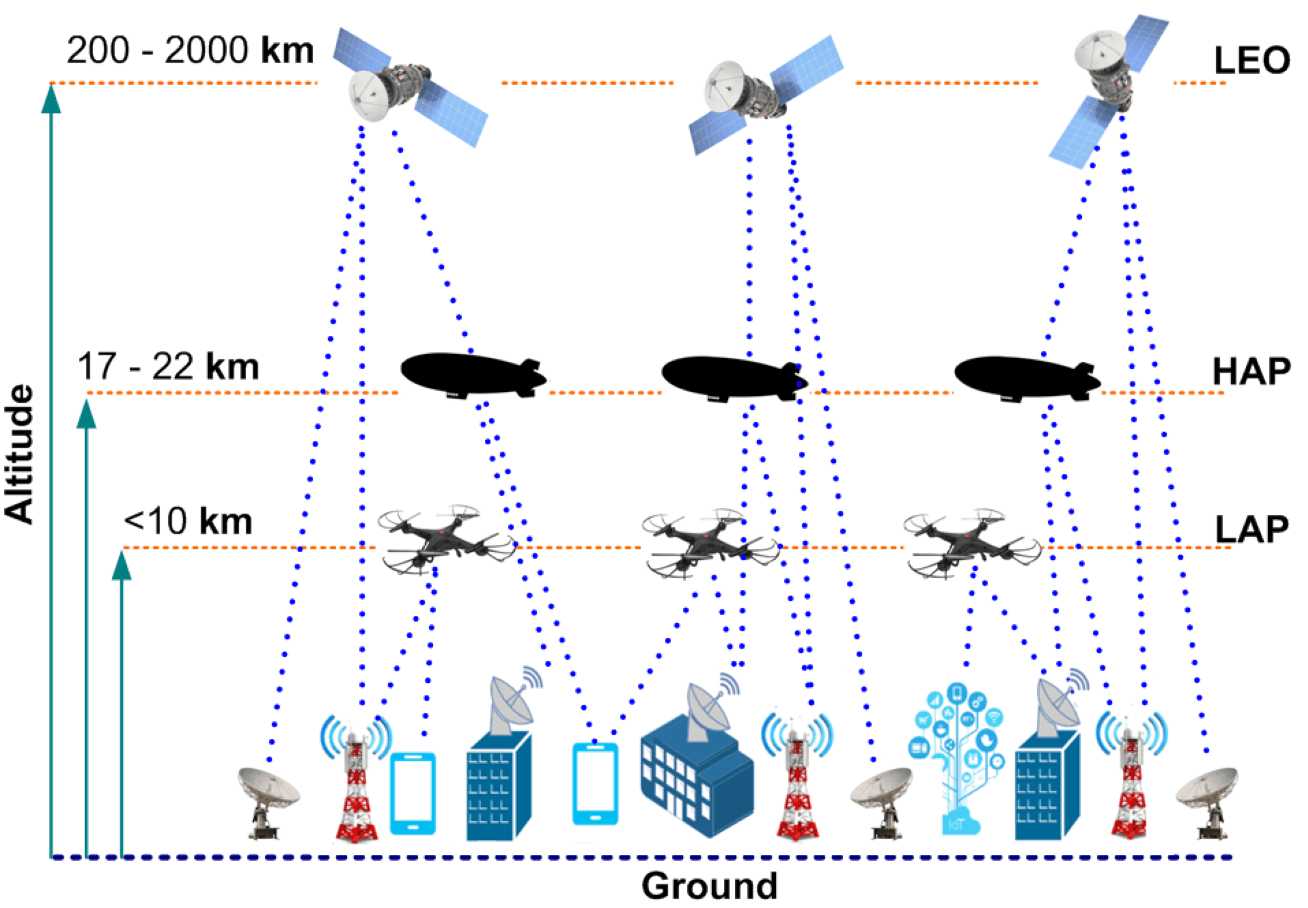The image depicts a colorful and detailed diagram illustrating the altitude range of different communication signals and devices. On the left, a vertical axis labeled "Altitude" is marked with three distinct green arrows, each pointing to significant altitude levels. 

At ground level, indicated by a dashed black horizontal line labeled "Ground," various icons represent satellite dishes, cell phone towers, and mobile phones. These ground-based devices are able to communicate with drones and other low-altitude platforms (LAPs) at altitudes less than 10 kilometers, marked by an orange dashed horizontal line. 

Further up, at an altitude range of 17 to 22 kilometers, labeled as "HAP," three blimps or high-altitude platforms are depicted floating horizontally, with their signal range extending downward to the ground. 

The highest marked altitude range is 200 to 2,000 kilometers, where low earth orbit (LEO) satellites are illustrated. Blue dotted lines originating from these satellites show the communication paths extending back to Earth.

Blue circular symbols and dotted lines illustrate the connectivity between various devices and platforms, demonstrating the layered structure of modern communication systems stretching from ground level to high orbital altitudes.